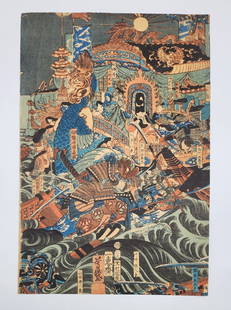The image depicts a complex and abstract artwork dominated by a structure that likely represents a building or possibly a boat, situated in the center. The image's lower resolution and busy composition make details challenging to discern. The predominant colors are various shades of blue, gold, beige, orange, yellow, green, brown, and gray. The central structure features a distinguishable roof adorned with possibly flagpoles and banners in gold and blue hues. 

At the top right of this structure, a bird or an abstract animal figure appears perched on the dark roof. The central doorway is framed with a goldish design reminiscent of flames or sun rays. Below, walkways or bridges extend from the structure, suggesting connectivity to other parts or leading out of the frame toward the right, over what seems to be dark grayish-green water.

The left side of the image includes additional structures in the water, complemented by vertical banners that appear to display Chinese characters. The scattered elements on the walkways and bridges in the center likely depict abstract figures or faces, enhancing the impressionistic quality of the artwork. The stormy gray background behind the central structure and other foreground elements suggests a tumultuous atmosphere.

Overall, the image conveys an intricate and storied scene of a structure on water, possibly of Asian origin, as indicated by the Asian writing and stylistic elements. This multifaceted depiction is rich in textures and colors, evoking a sense of mystery and depth.